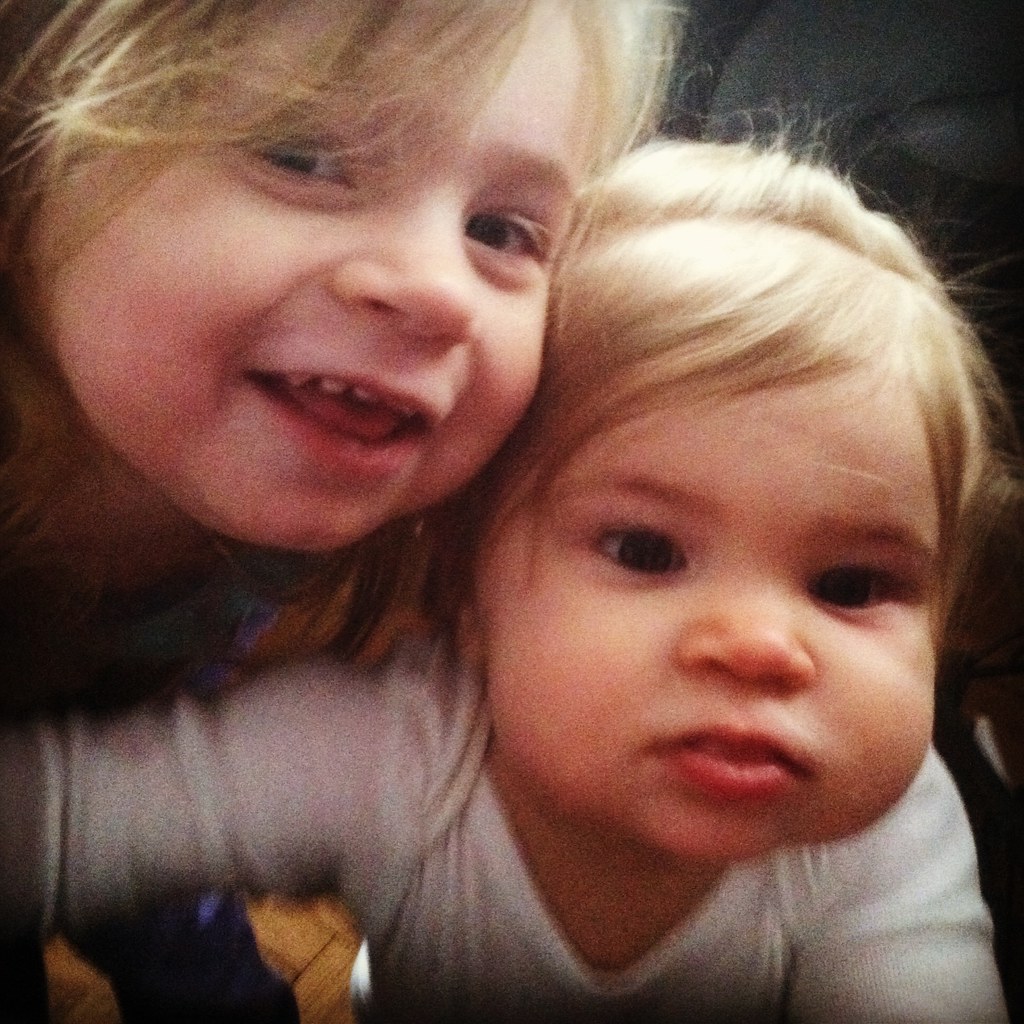This photograph features a close-up image of two young girls, possibly sisters, with their faces close together—cheek against forehead, or side of the head—creating an intimate and affectionate pose. The younger girl on the right appears to be around two or three years old, with blonde hair brushed away from her face. She has chubby cheeks and ambiguous eye color, likely green or brown, and is dressed in a white shirt. The older girl, positioned slightly above and to the left, showcases an open-mouthed smile, revealing a few small teeth, and is gazing joyfully at the camera. She also has blonde hair, albeit partially obscuring her left eye. She is dressed in what seems to be denim, possibly blue jeans or a blue overall. Their identical blonde hair and similar facial features suggest a strong familial resemblance. The background hints at a black couch, adding context to the cozy, indoor setting.